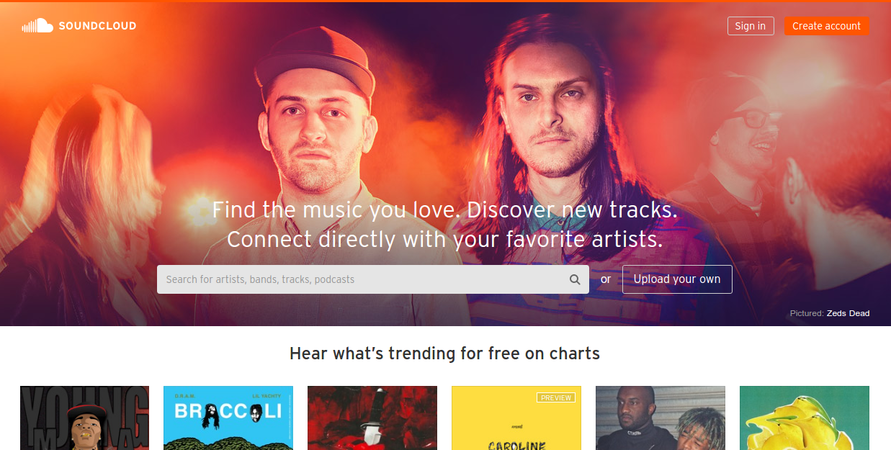This screenshot from SoundCloud features a hero image of two young men and a muted, orange-hued background. The man to the left sports a flat-brim baseball cap over his closely-cropped hair, accompanied by stubble and a button-down shirt. Beside him, another man, possibly in a polo shirt, has long hair parted in the center, a scruffy face, and looks slightly blurred.

The image overall is suffused with an orange haze and features light leaks, adding to the vintage atmosphere. An orange overlay covers parts of the screen, and glimpses of people can be seen in the background. SoundCloud's logo is positioned in the upper left corner, followed by 'Sign in' and 'Create account' options. Central white text on the image promotes SoundCloud's offerings: "Find the music you love, discover new tracks, connect directly with your favorite artists.” Below this text is a search field marked "Search for artists, bands, tracks, podcasts," along with a button for uploading your own content.

Prominent just below this is the section titled "What's trending for free on charts," showcasing six trending albums. Although the album covers are partly obscured, they vary in color and style, including combinations of black, blue, red, yellow, and green hues with various photographic elements.